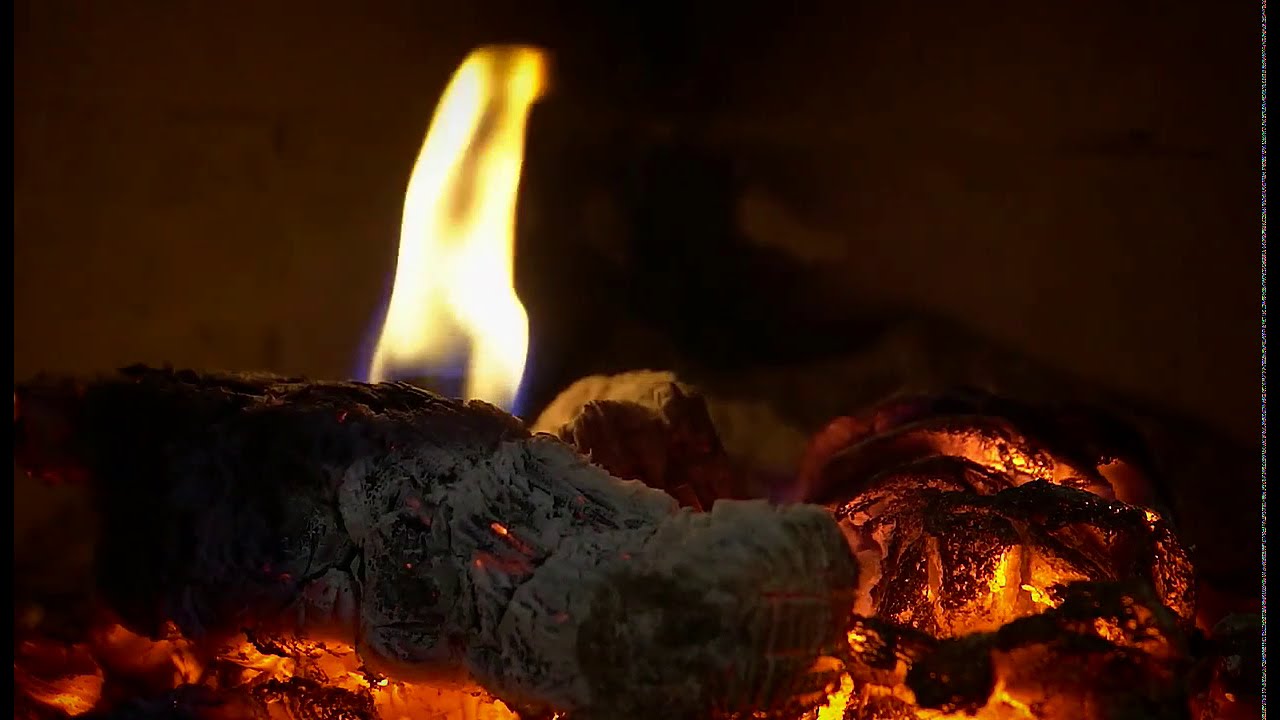This image is a close-up of a roaring fire, possibly in a fireplace or outdoor fire pit. The main focus is a charcoaled wooden log that extends horizontally from the left side, stopping just past the center of the frame. The log is extremely charred, especially on the left, where it appears almost black. More vibrant hues of red and orange embers surround the log at the bottom and to the right, while a strong, vivid flame rises from its center. This flame exhibits a spectrum of colors: a blue base transitioning to white, then yellow, with bursts of yellow and orange fire glowing intensely. The background is dark, with dim orange and brown tones, punctuated by a concentrated black area in the middle. The scene radiates intense heat, capturing the transformative process of the wood turning to ashes, with gray ash evident in the foreground. Overall, the image vividly portrays the dynamic interplay of fire and embers, enveloped in an aura of warmth and combustion.